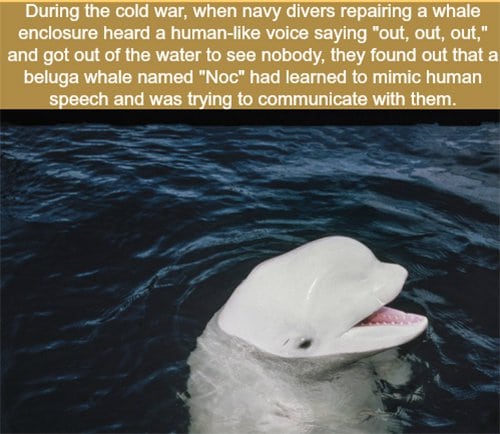The image features a bright white beluga whale with a pink mouth and black eyes, emerging from dark blue ocean water with its mouth open. At the top of the image, white text on a beige background reads: "During the Cold War, Navy divers repairing a whale enclosure heard a human-like voice saying 'out, out, out, out.' When they got out of the water to investigate and found nobody, they discovered that a beluga whale named Nock had learned to mimic human speech and was trying to communicate with them." The water dominates the lower part of the image, and the whale is positioned towards the bottom right. The overall colors in the image include white, blue, brown, and a touch of pink.